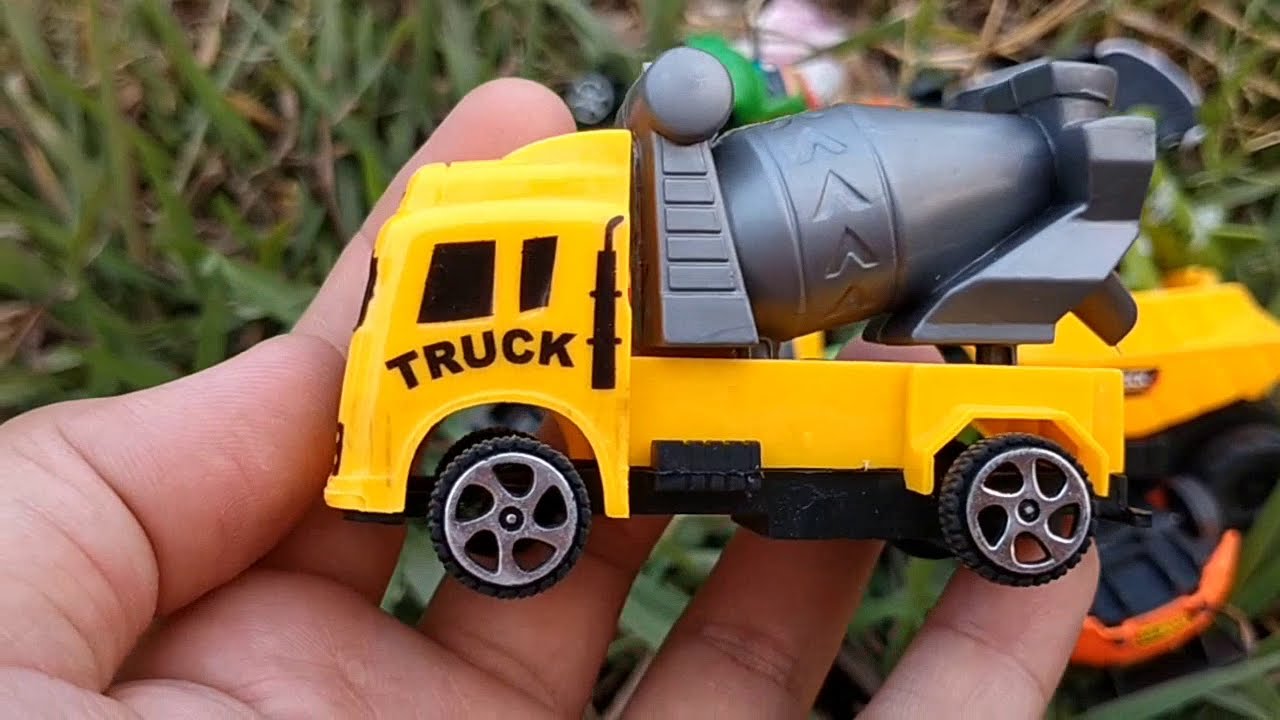The image depicts an outdoor, daytime setting, possibly in someone's backyard, with a grassy background. Central to the image is a yellow toy cement truck, held by a man's hand emerging from the bottom left corner. The toy truck is positioned sideways with the front facing left. On the side of the truck, near the driver's door, is the word "truck" written in black lettering. The truck features two windows, a smokestack pipe, black wheels with silver rims, and a silver cement mixer adorned with upside-down 'V' shapes as a decorative feature. In the background, partially obscured and slightly blurry, there are additional toys, including an orange toy car overturned on the grass and a glimpse of another yellow vehicle. The overall image is bright, clear, and richly colored, highlighting an everyday moment of a person picking up children’s toys from the lawn.